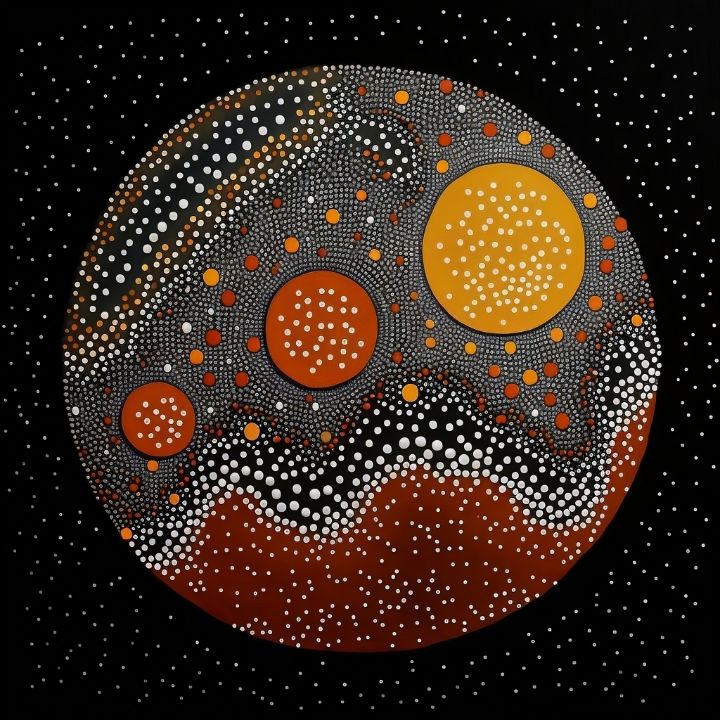This mesmerizing painting depicts a celestial scene centered around a large, intricately detailed circle set against a pitch-black background speckled with countless tiny white dots, reminiscent of stars in the vastness of space. The large circle, resembling a distant planet, displays a complex array of dot art with hundreds, if not thousands, of small dots varying in density to create rich textures and gradients. Dominating this planetary form are three prominent circles: a mustard yellow circle positioned in the upper right, and two darker orange circles of different sizes situated lower to the left, one with lighter polka dots. These circles are artfully layered, with geometric shapes and vivid colors—white, orange, deep rust red—harmoniously integrated amidst the sea of dots, evoking the feeling of wild and uncharted territories in the cosmos. This artwork is both a visual intrigue and a testament to the meticulous craft behind dot art, encapsulating a sense of cosmic wonder.